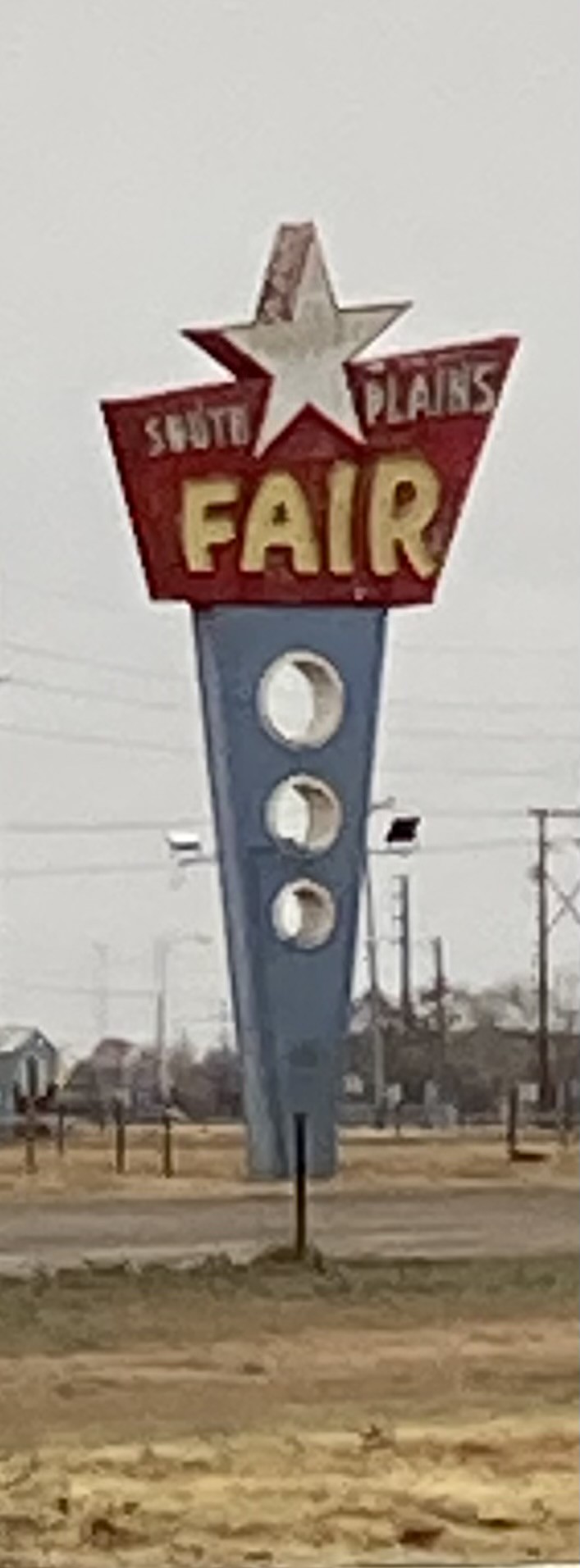In this image, a distinctive sign stands prominently in the distance. The foreground features a patch of dirt, transitioning from a yellowish hue at the front to a deeper brown further back. Cutting horizontally across the middle of the scene is a gray street, providing a sharp contrast to the earthy tones below.

The focal point of the image is a vertically positioned, blue-tinted sign resembling the shape of a pizza slice. The sign is distinctly marked by three circular holes, diminishing in size from top to bottom, all outlined in gray with white hollow centers. At the top of the sign, in front of a red background, the words "South Plains Fair" are emblazoned, crowned by a whitish-gray star.

In the background, a series of trees and several telephone poles are visible, adding depth to the scene. The sky above completes the composition with a light gray hue, enhancing the overall muted yet detailed palette of the image.